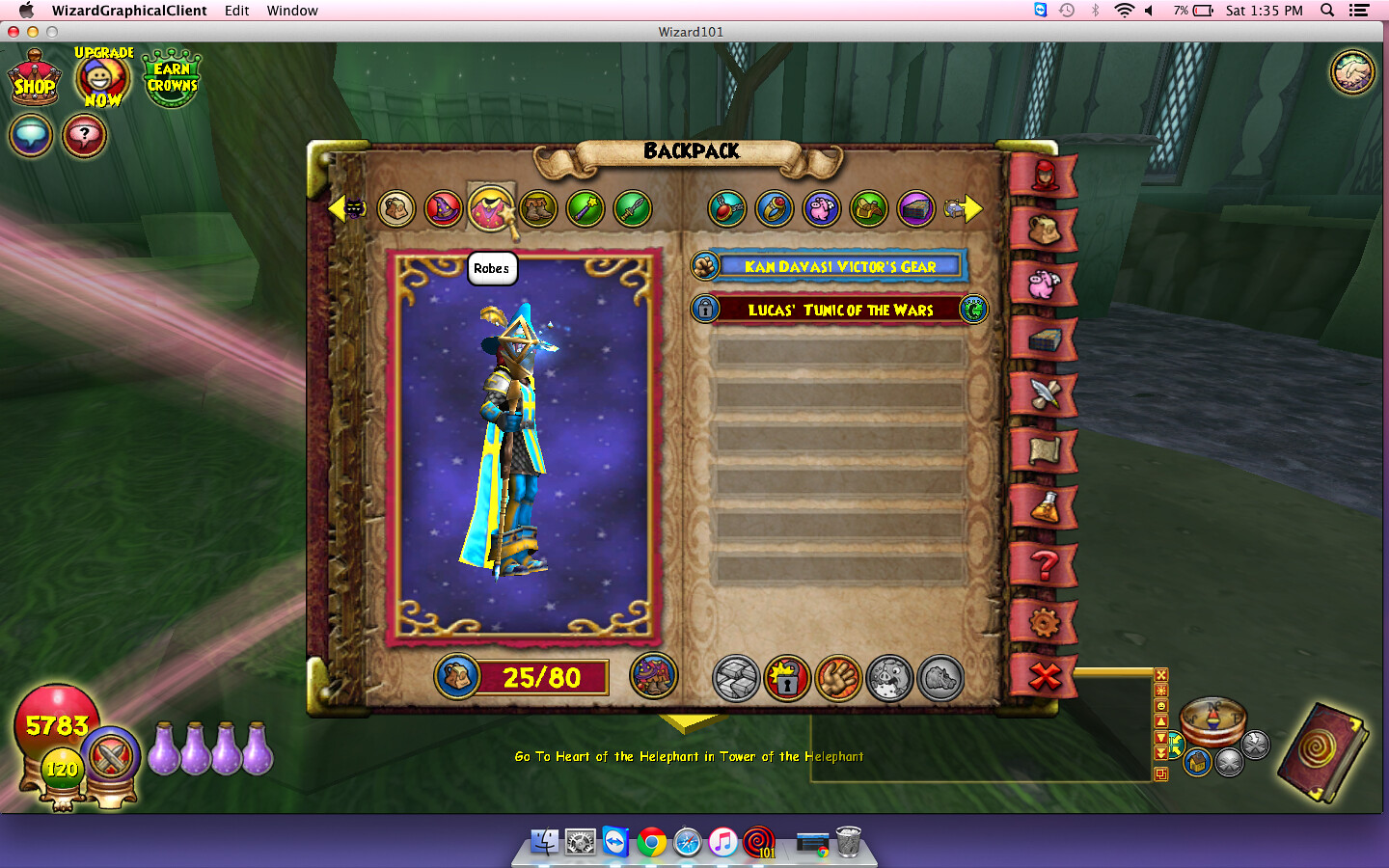The screenshot depicts a windowed role-playing game (RPG) interface on a Macintosh computer. The game window is positioned between the top taskbar, labeled "Wizard Graphical Client," and the Mac dock at the bottom, which displays various icons such as Safari and iTunes. The game screen shows an animated background of a room, with a central box labeled "Backpack." Inside the box, a futuristic warrior character is displayed. The interface features a numerical indicator of "25/80" for character upgrades, suggesting that the character is still in the early stages of development. On the left side of the screen, there are tabs for different in-game options, such as changing outfits or weapons. Additionally, a quest directive at the bottom reads, "Go to the heart of the Hyrule Port in Tower of the Temple Heart," and the player's score is shown as 5,783.